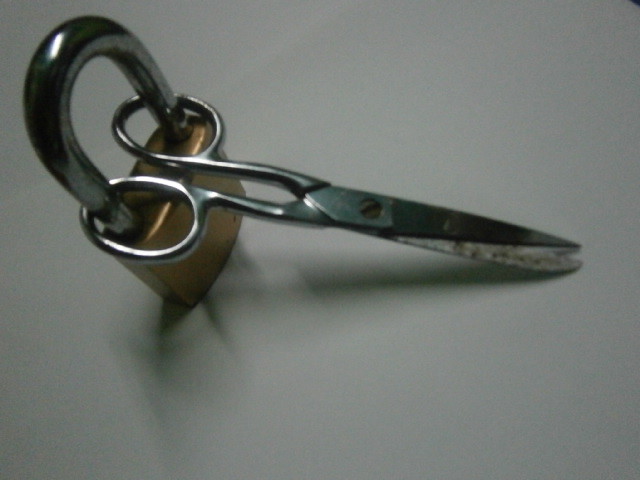This photograph features a large brass-colored padlock with a silver, U-shaped, steel locking mechanism securing an old, slightly rusted pair of metal scissors. The padlock, which operates with a key, has its thick, horseshoe-shaped shackle passed through the circular finger holes of the scissors. The scissors, displaying patches of rust and debris on their blades, are mostly closed and locked tightly by the padlock. The scene is set against a gray background, casting shadows of both the lock and scissors on the surface.